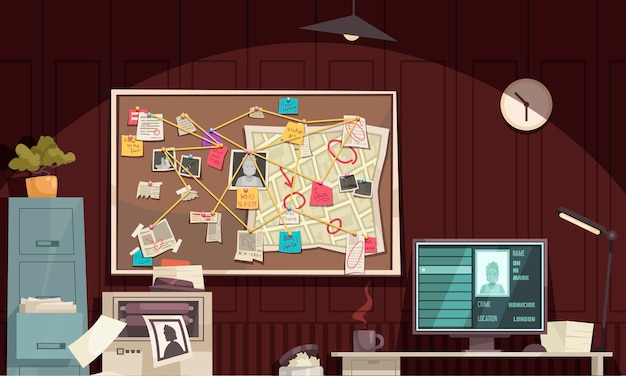This animated, digitally drawn image features a detailed interior scene set against a maroon-colored wall with vertical patterns, resembling inbuilt wardrobes or closed shelves. A white clock with a circular face, displaying the time as ten minutes to six, is mounted on the wall. From the ceiling hangs a lamp with a white bulb and gray lampshade, casting light on the room's contents. Prominently displayed is a large rectangular notice board with a white border and brown background, adorned with various photographs, newspaper clippings, and a map, interconnected by yellow string.

Below the notice board sits a cluttered desk, featuring a flat-screen computer monitor displaying a picture and data, a coffee mug emitting steam, and a lamp providing additional light. To the side of the desk stands a blue, steel-gray vertical shelf that includes a partially open drawer with white papers spilling out. Atop this shelf is a plant with green leaves in a yellow vase. A white printing machine on the floor next to the shelf ejects paper, contributing to the scene's sense of animated chaos. A filled wastepaper basket completes the busy, detailed setting.